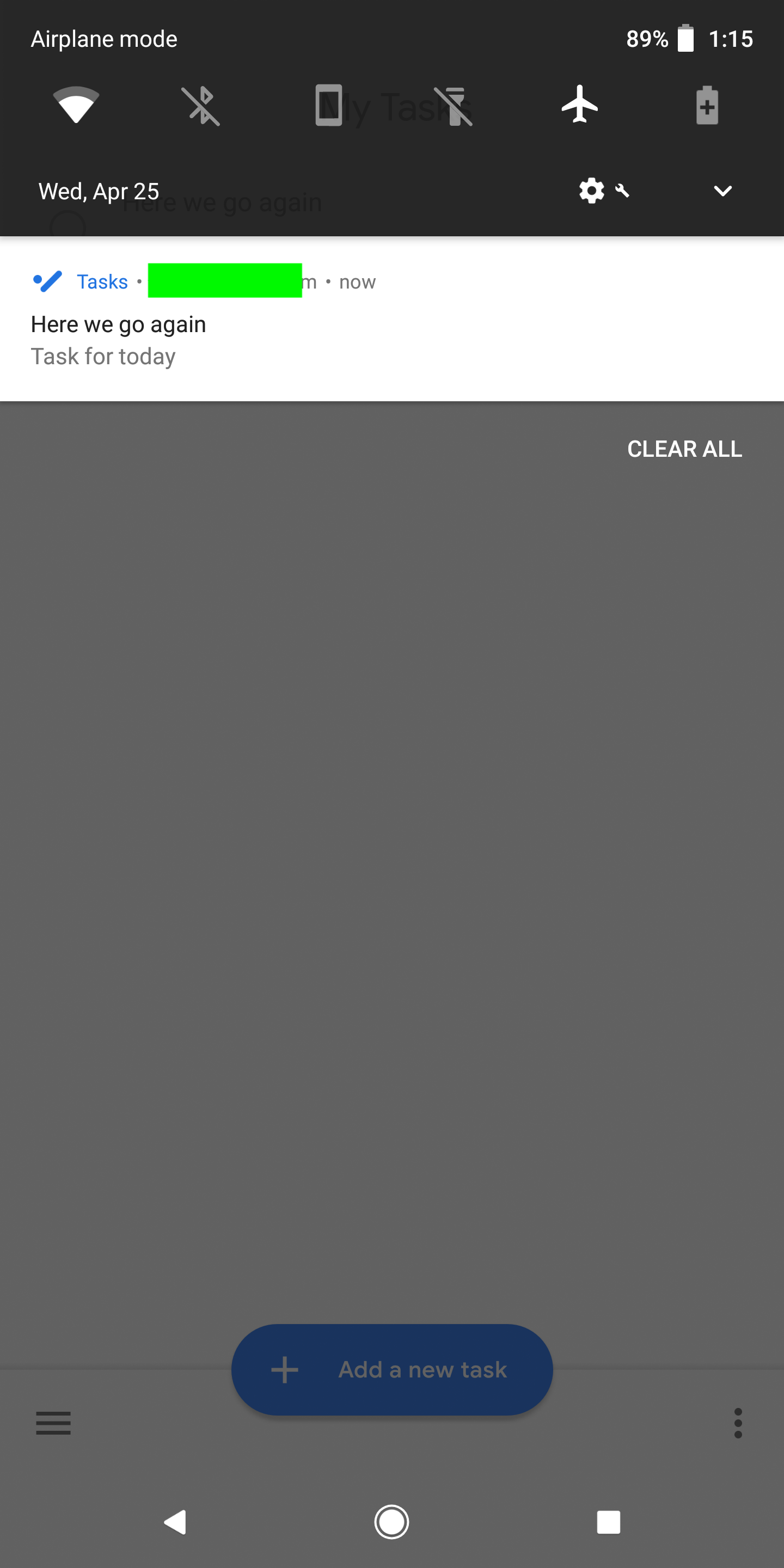This is a detailed screenshot from a person's cell phone. The topmost section of the screen features a black banner displaying the status indicators: "Airplane Mode," 89% battery, and the time "1:15." In sequence from left to right, the icons shown are Wi-Fi, Bluetooth, a crossed-out flashlight, airplane mode, and battery. Below this banner, the date "Wednesday, April 25th" is prominently displayed.

The main section of the screen is titled "Tasks," and features an area obscured by a green rectangle, presumably to redact sensitive information. The text beneath the redaction reads, "Here we go again. Tasks for today."

A long, grayed-out vertical rectangle appears below this section, with "Clear All" in white letters positioned at the top of it. At the very bottom of the screen is a blue oblong button containing a white plus sign and the text "Add a new task" in white letters.

In the bottom navigation area, three symbols are visible: a white arrow pointing to the left, a white circle, and a white square. The image itself is taller than it is wide, with no photographic elements. The screenshot contains no people, animals, birds, plants, flowers, trees, or buildings.